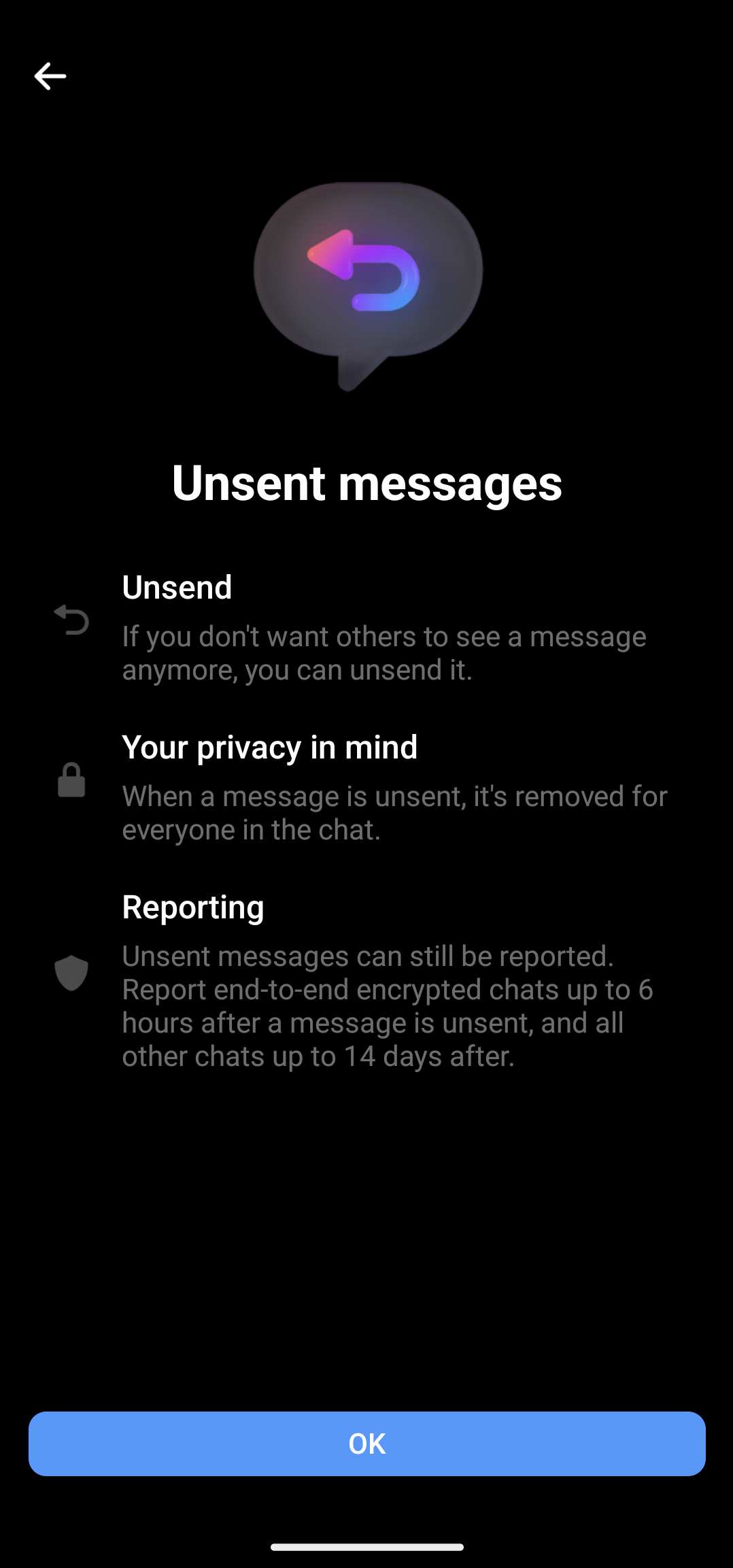This is a detailed caption for the provided image:

---

The image is a portrait-oriented screenshot of a phone's settings menu, approximately two to three times taller than it is wide. The background is predominantly black, creating a high-contrast setting for the text and icons displayed on the screen. In the upper left-hand corner, there is a white back arrow, indicating a navigational option to return to the previous menu.

Centrally positioned at the top of the screen is a semi-transparent, grayish text bubble featuring a vibrant icon. This icon consists of a looped arrow that starts at the bottom, forming a U-shape with a left-pointing arrowhead at the top, colored in gradients of pink, purple, and blue.

Beneath this icon is a bold white header reading "Unsent Messages". Directly underneath, in smaller white text, it states "Unsend", accompanied by a gray descriptive line: "If you don't want others to see a message anymore, you can unsend it." Next to this explanatory text is a reverse arrow icon, reinforcing the 'unsend' action.

Further down the screen, there is a lock icon followed by the phrase "Your Privacy in Mind." The adjacent gray text explains, "When a message is unsent, it is removed for everybody in the chat." This reassures users about the privacy measures in place.

Continuing downward, another white header titled "Reporting" is present, complemented by a gray shield icon to its left. The associated description details, "Unsent messages can still be reported. Report and send encrypted chats up to six hours after a message is unsent, and other chats for up to 14 days after."

At the bottom of the screen is a long rectangular blue button with rounded edges, saying "OK" in white font. Directly beneath this button is a thin, white horizontal line, marking the end of the informational section.

---

This detailed description includes all visual and textual elements captured in the screenshot, providing a comprehensive understanding of the image's content and layout.